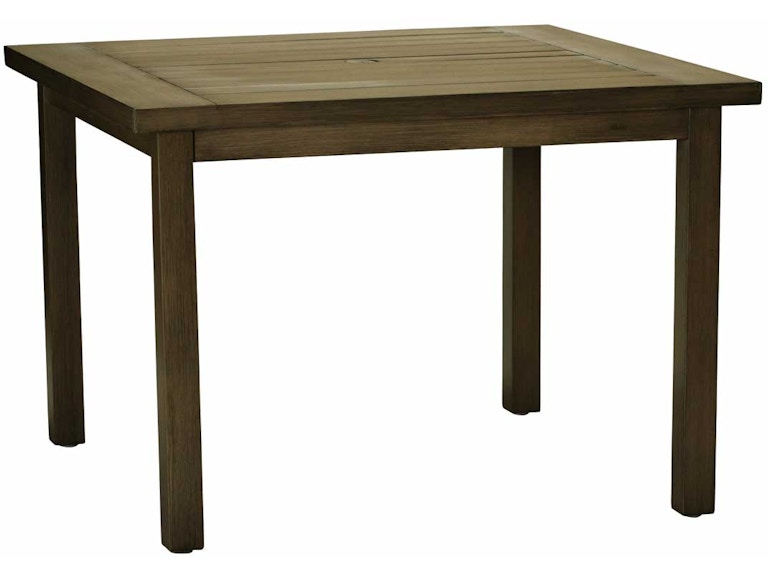This image features a simple, rectangular wooden table set against a completely white background, emphasizing its product-like presentation. The table is composed entirely of dark brown wood and has four straight legs that are rectangular prisms extending down to the ground, equally spaced from each corner. The tabletop consists of two wider wooden planks running along the shorter ends, with several narrower but longer pieces of wood situated perpendicularly between them. There is a noticeable hole in the center of the table, possibly intended for an umbrella. The table's surface is flat and lacks any glossy finish, suggesting it might be designed for exterior use. The overall simplicity and plain design of the table give it a rustic aesthetic suitable for various settings.